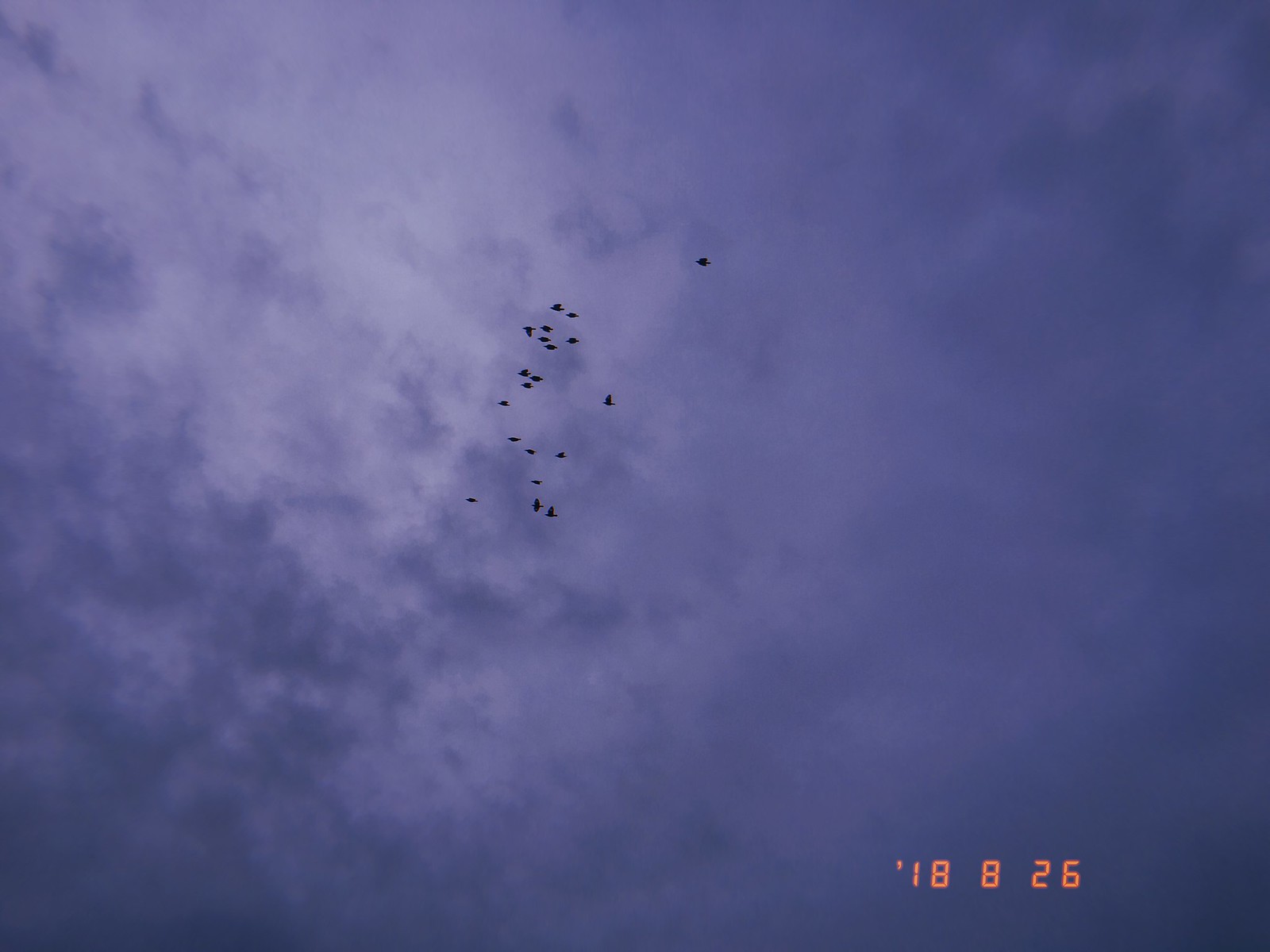This photograph captures a dramatic, overcast sky with varying shades of dark gray and hints of dark blue and purple. The majority of the sky is dominated by dark clouds, particularly concentrated in the bottom left, bottom right, and top right corners, while the clouds in the top left are slightly lighter. Central to the image is a flock of approximately 20 birds, appearing as small, black specks against the slightly lighter clouds in the middle. Notably, one bird is slightly ahead of the main group on the right side. Adding an interesting element, the bottom right of the image features an orange digital timestamp '18-8-26' with an apostrophe preceding the 18, marking the date the photograph was taken. Despite its high quality, the image has a slightly grainy texture.